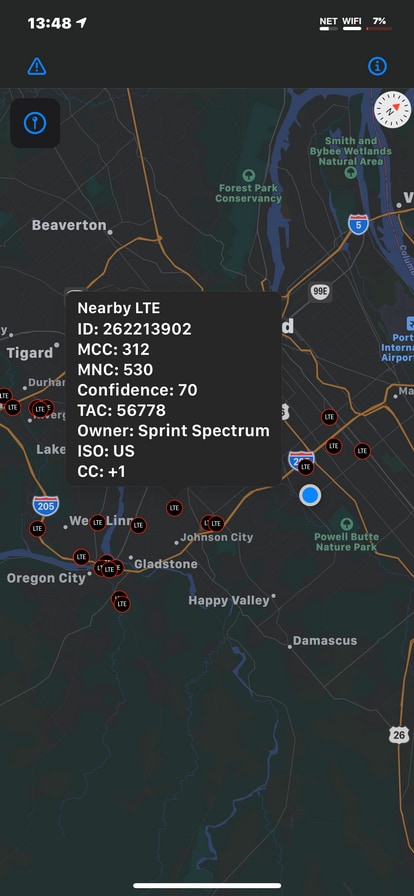The image displays a detailed screenshot taken from a smartphone, showcasing a comprehensive map interface. The map itself is rendered in a dark gray color scheme, highlighted by blue lines representing rivers or streams that crisscross the terrain. Prominent yellow paths indicate major roads, while lighter gray lines delineate smaller streets and thoroughfares. White text labels various cities and regions on the map, providing clear geographical markers.

Centrally positioned on the map is a large, dark gray text box, square in shape, containing white text that reads: "Nearby LTE ID" followed by various data points including an MCC number, an MNC number, a confidence number, a TAC number, the owner's name, the label "ISO US," and "CC +1." 

At the top of the screen, the status bar features the time "13:48" displayed in white text on the top left, while the top right shows the network status "Net Wi-Fi" and the battery level at "7%," along with a white navigation or compass icon encircled. This status bar sits against a dark gray or black background, adorned with blue navigation buttons.

The bottom of the image is bordered by a white bar that stretches across the screen. The photo itself is characterized by its vertical, narrow rectangle shape, with the longer sides extending left to right. The detailed elements and color contrasts create a functional, visually cohesive tool for navigation and information display.